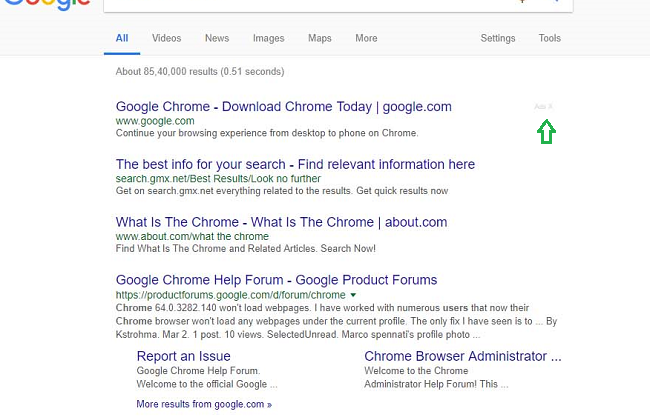A Google search results page is displayed, although the top part is cut off. The familiar multicolor Google logo is partially visible at the upper portion, showcasing its iconic rainbow hues. Directly beneath the logo is the search bar, empty and awaiting input against a stark white background. Above this, the navigation menu sits on a light gray strip, featuring tabs labeled All, Videos, News, Images, Maps, and More, with the "All" tab highlighted to indicate the current selection. The results area starts with a statement that reads "About 85 million results," implying a high number of potential matches found for the query.

The first search result is a link to Google Chrome, hinting that the user may have been searching for a web browser. The top result prominently displays this, suggesting it as the best option according to Google. The page text appears in black, with the URLs presented in green and the clickable links underlined in blue. Subsequent results include "Google Chrome, the best info for your search" from searchgmx.net, "What is the Chrome" from about.com, and "Google Chrome Help Forum" located in the Google Product Forums. This selection of links provides various resources related to Google Chrome, ranging from general information to specific user support.